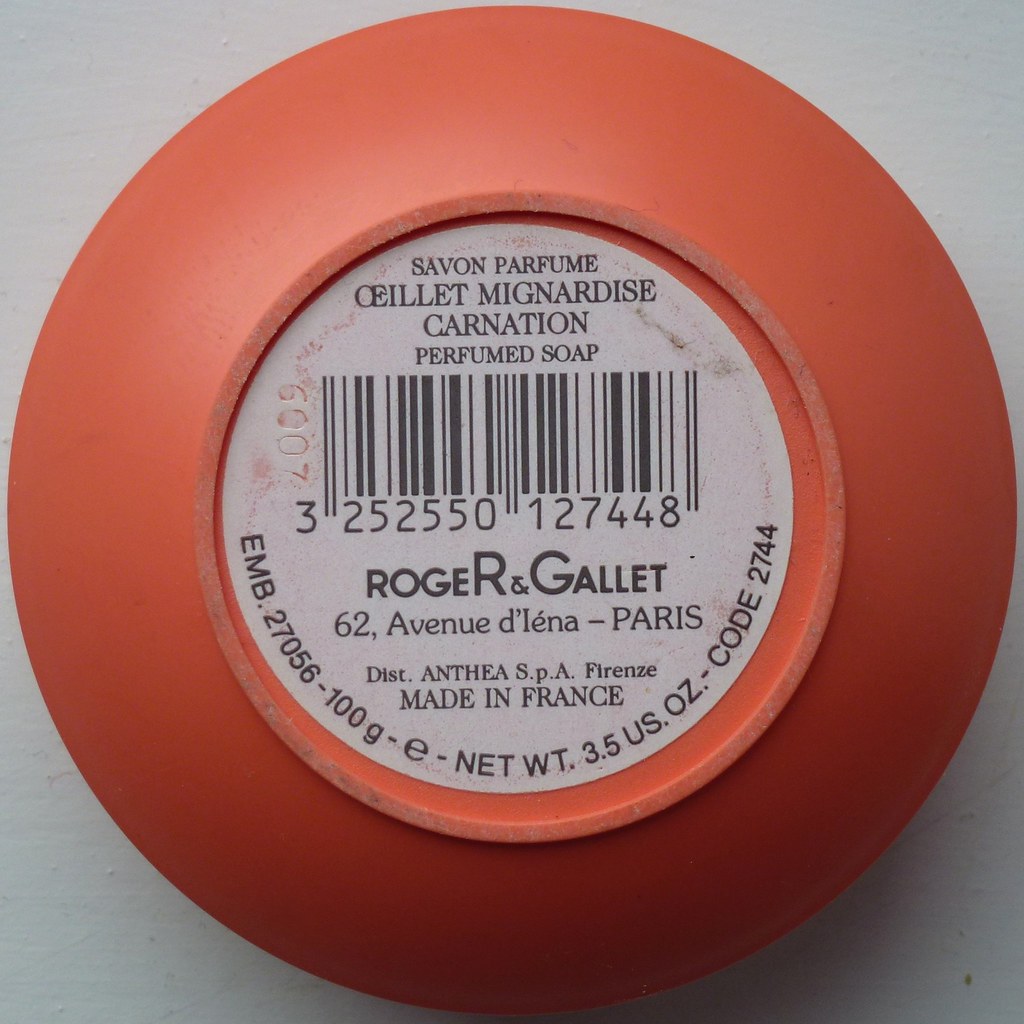In the image, there is a single, centrally positioned circular object, possibly the bottom of a bowl or a container, prominently featured against a greyish or white background that is visible only at the corners (upper right, upper left, lower right, and lower left). The object is predominantly orange with a white sticker in the middle, bordered by an outlined circle. The sticker contains detailed text: at the top, it reads "Savon Parfumé" followed by "C-E-I-L-L-E-T M-I-G-N-A-R-D-I-S-E", then "Carnation" and "Perfumed Soap" in smaller letters. Below this, there is a barcode with "Roger and Gallet" in large black letters, an address mentioning "Avenue D'Elena, Paris, District Athena, SPA, Forenz", followed by "Made in France". Curved along the bottom from middle left to middle right are additional details including net weight and a code. The setting appears to be indoors or perhaps a stock image for soap sales, with colors primarily grey, orange, white, black, and tan.